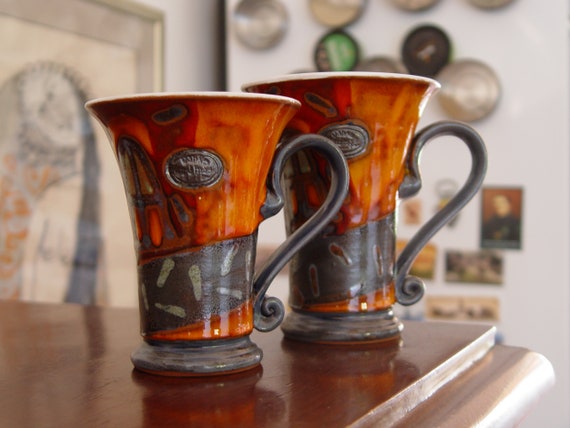The image depicts two antique-style ceramic mugs prominently displayed on the corner of a dark, polished wooden bar or countertop. The mugs are bell-shaped, narrower at the base and flaring out towards the top. They feature a dark black base and matching handle, while the main body of the mugs has a wood-grain finish, simulating the appearance of a tree trunk. A black band encircles the middle of each mug, adorned with an intricate design. Close inspection reveals an "A" engraved on both mugs, which also seem to have a ribbon-like band with little bottles around it and sit on a small podium-like base. 

In the background, the image offers a glimpse into what appears to be a creatively decorated interior space, possibly someone's home. To the left, a white wall hosts a large, gold-framed abstract painting that seems to depict a nude woman with very long hair, tilting to one side, with a purple and orange blanket next to her. The wall also includes other artwork, including a piece that might be a Van Gogh reproduction. Additionally, a section of a wall with various records and more paintings is visible, contributing to the artistic ambiance of the setting.